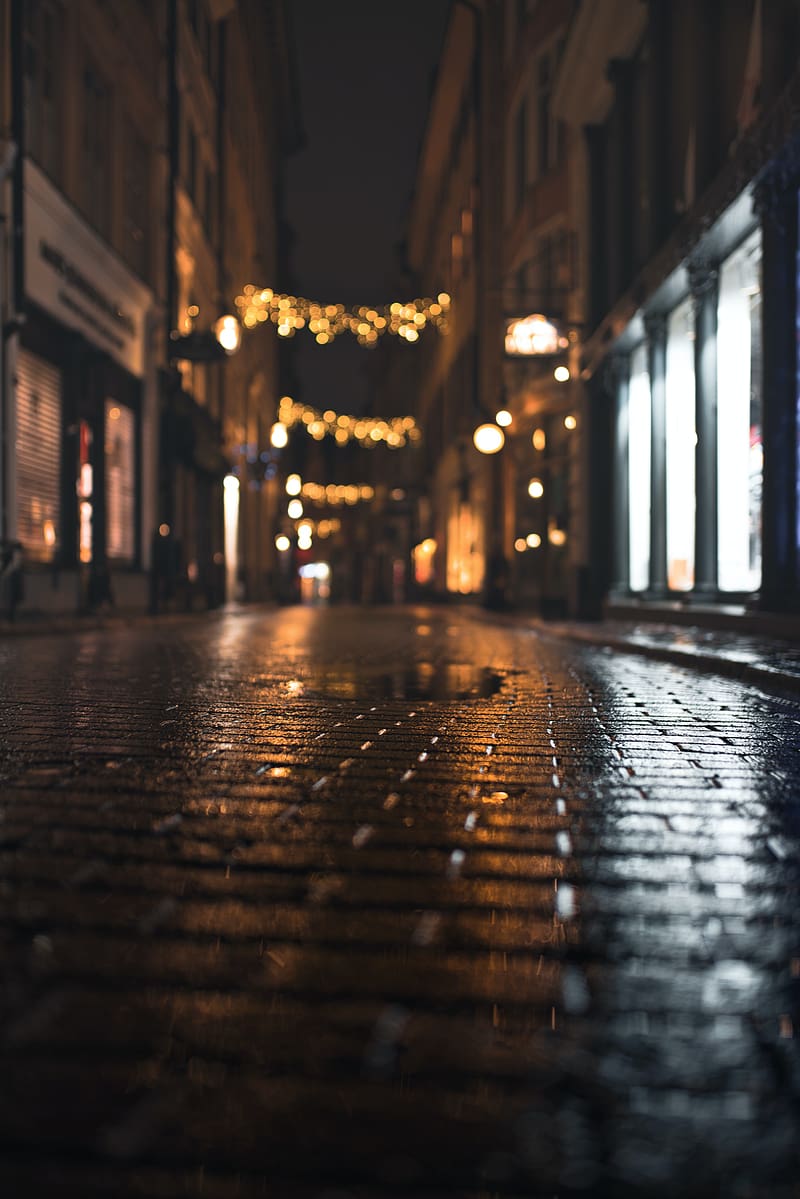The image depicts a deserted brick or cobblestone street in a city at night, evoking a melancholic atmosphere due to its emptiness. The street, glistening with moisture, reveals a shiny surface with a couple of puddles reflecting the surrounding lights. The buildings on either side of the street are closely spaced, constructed from bricks and stone, reminiscent of an older era, possibly the late 1800s. Despite the buildings' historical appearance, it's a modern photograph. Strings of white Christmas lights, mimicking icicles, hang in rows across the street, extending into the distance and adding a serene, festive touch to the scene. Some buildings feature illuminated floor-to-ceiling windows, likely showcasing displays, although the exact details are obscured due to blurring. Other storefronts are closed for the night, with protective metal shutters pulled down. The sky is pitch black, suggesting it is very late, perhaps with fog or clouds further darkening the atmosphere. The overall color palette consists of dark browns, grays, and blacks, with the bright, vivid lights providing the primary contrast.